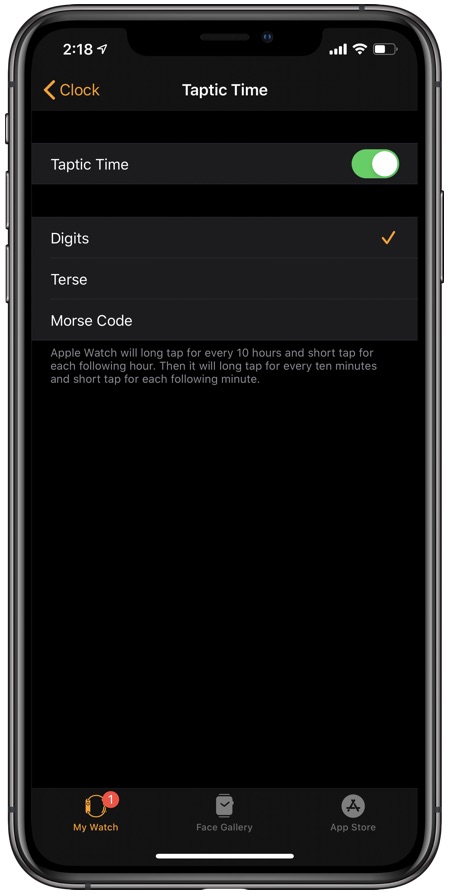The image showcases a modern iPhone without a cover, displaying its home screen. The phone is connected to Wi-Fi and has a visible battery icon on the top right corner, with the current time shown as 2:18 PM on the top left. The screen is focused on the "Taptic Time" settings, evident from the title at the top.

The "Taptic Time" feature has a toggle button, which is currently turned on. Below the toggle, there are three options for the Taptic Time feedback style: Digits, Terse, and Morse Code. The "Digits" option is selected, as indicated by a checkmark, while the other two remain unchecked. 

On the left side of the screen, there is an arrow pointing left, along with a clock icon, indicating a navigational option within the settings. 

Towards the bottom of the screen, an illustration of an Apple Watch appears with a small notification badge showing the number "1". Below this, there are options labeled "Face Gallery" and "App Store." The interface suggests that these settings are customizable options for the Apple Watch's Taptic Time feature, which provides haptic feedback to indicate the time.